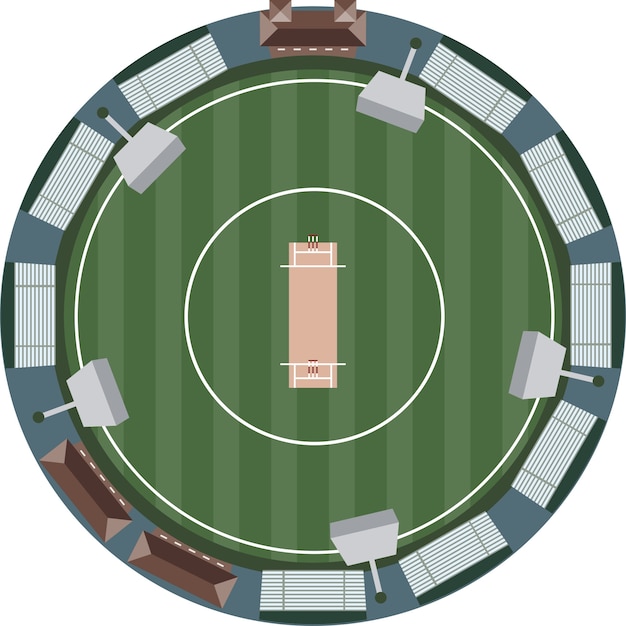The image depicts a detailed diagram of a circular stadium with a field at its center, surrounded by bleachers and distinct sections. The bleachers, forming the outer ring, have a mix of white and light gray colors with blue accents at their tops. Some lines of gray intersperse the bleachers, contributing to their tiered appearance. Additionally, there are three rectangular, maroon-colored roof segments, possibly housing for announcers or equipment, arranged around the stadium's perimeter.

The field showcases alternating light and dark green stripes, indicating different sections of the playing surface. Encircling the field are two distinct thin white outlines, marking the boundary lines. At the very heart of the field lies a tan or peach-colored rectangular court-like area. Centered on this court are two white goals or structures with red markings.

Around this central field, stadium lights on big posts are visible, hinting at their placement around the stadium. The ground beneath, possibly synthetic, mimics real grass with its green stripes, adding to the field's detailed design. Overall, the diagram meticulously illustrates various elements of a modern stadium setup, blending both practical and illustrative components.